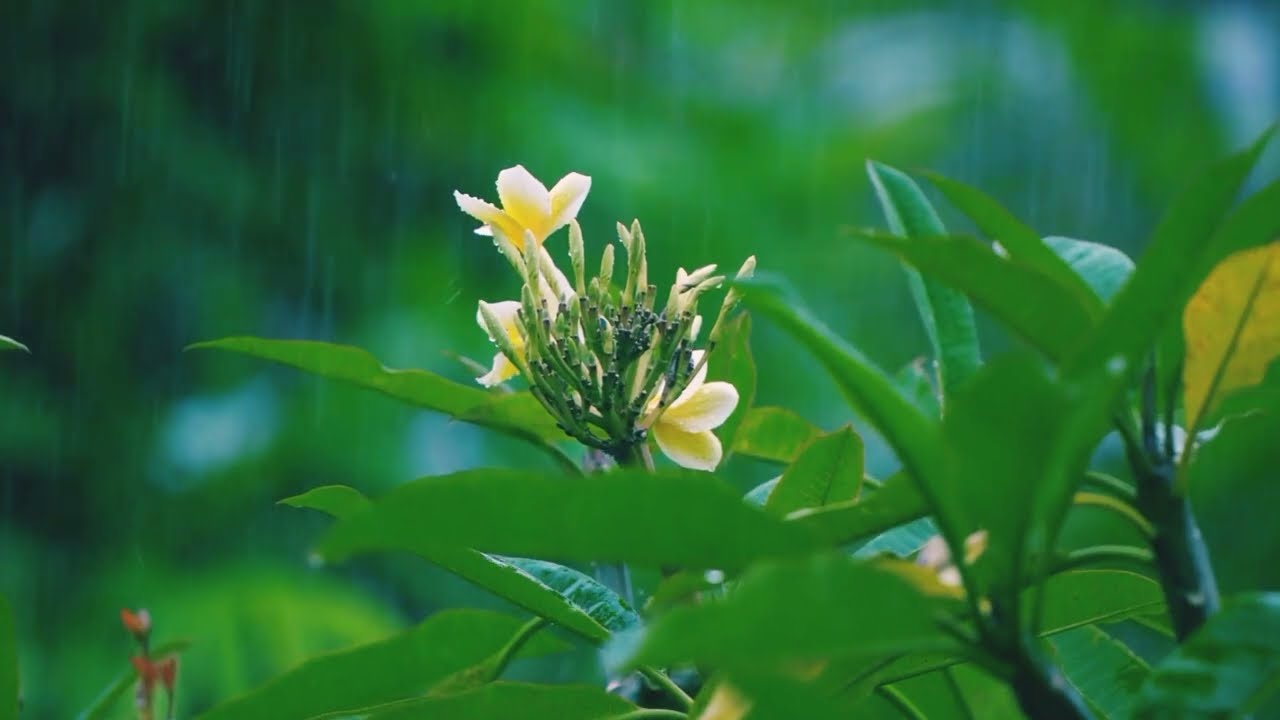The image is a highly detailed macro shot focusing primarily on a small bud at the center of a flower. This small bud is yellow with white-tipped petals, making it the focal point of the composition. Surrounding the central flower bud, the setting features a collection of green leaves, some of which have tiny buds with black tips. There is an orange nub visible in the bottom-left corner and a scattering of reddish flower elements. The right side of the image showcases various green stems and foliage with small green leaves. The background is notably blurred with a strong bokeh effect, highlighting the shades of green, orange, yellow, brown, black, and white. The overall scene is set outdoors in what appears to be a rainstorm, as evidenced by vertical streaks of water descending through the image. There are no text or people present, emphasizing the solitary beauty of this nature-focused scene.